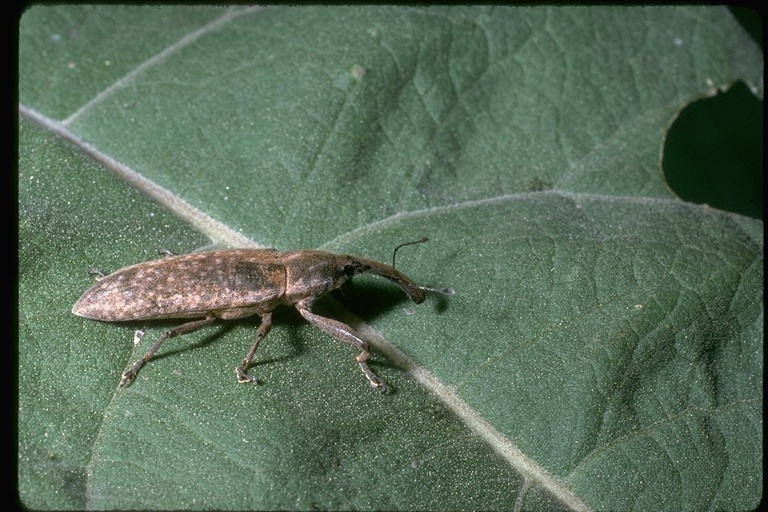A detailed photograph depicting a velvety, dark green leaf adorned with distinct beige veins. A weevil insect, brown with tiny beige speckles, is positioned toward the lower left of the image. It features a long, curved snout reminiscent of an anteater's trunk, six jointed legs, and two antennae extending from its snout. The leaf appears to have a black border on the right edge, enhancing the night-time atmosphere of the scene. A tear is visible on the top right corner of the leaf, adding to the intricate details captured in this highly realistic and representational photograph.